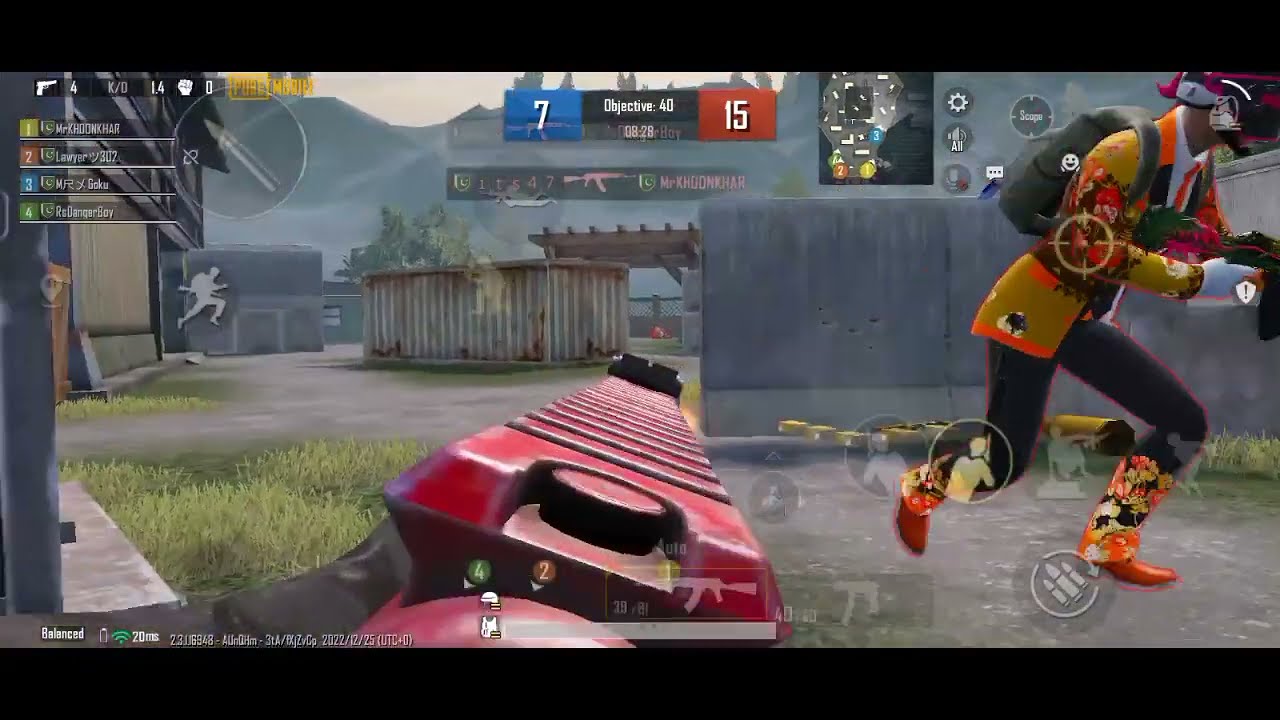The image depicts a scene from a first-person shooter video game, framed with thick black borders at the top and bottom. The player’s view includes the top part of a red-painted long gun with small black sights at the end, suggesting their in-game perspective. The foreground showcases a dirt pathway strewn with grass patches, alongside a concrete platform. A prominent gray concrete wall, shaped like an L, stands on the right side with more grass growing in front of it. Further to the right, a visually striking character is in mid-run towards the right edge of the image. This character wears distinctive flower-patterned orange and black cowboy boots, black pants, and an elaborate mustard-yellow jacket with orange trim and floral accents. They also sport a pink helmet, a black backpack, and are armed with a vividly colored green and pink gun. In the background, a rusty metal square structure and a larger brown structure are visible, with green mountains and clear skies beyond them. A mini-map and a score display indicating "Blue Team: 7 kills, Red Team: 15 kills" are situated at the top center of the image, underscoring the competitive nature of the game.